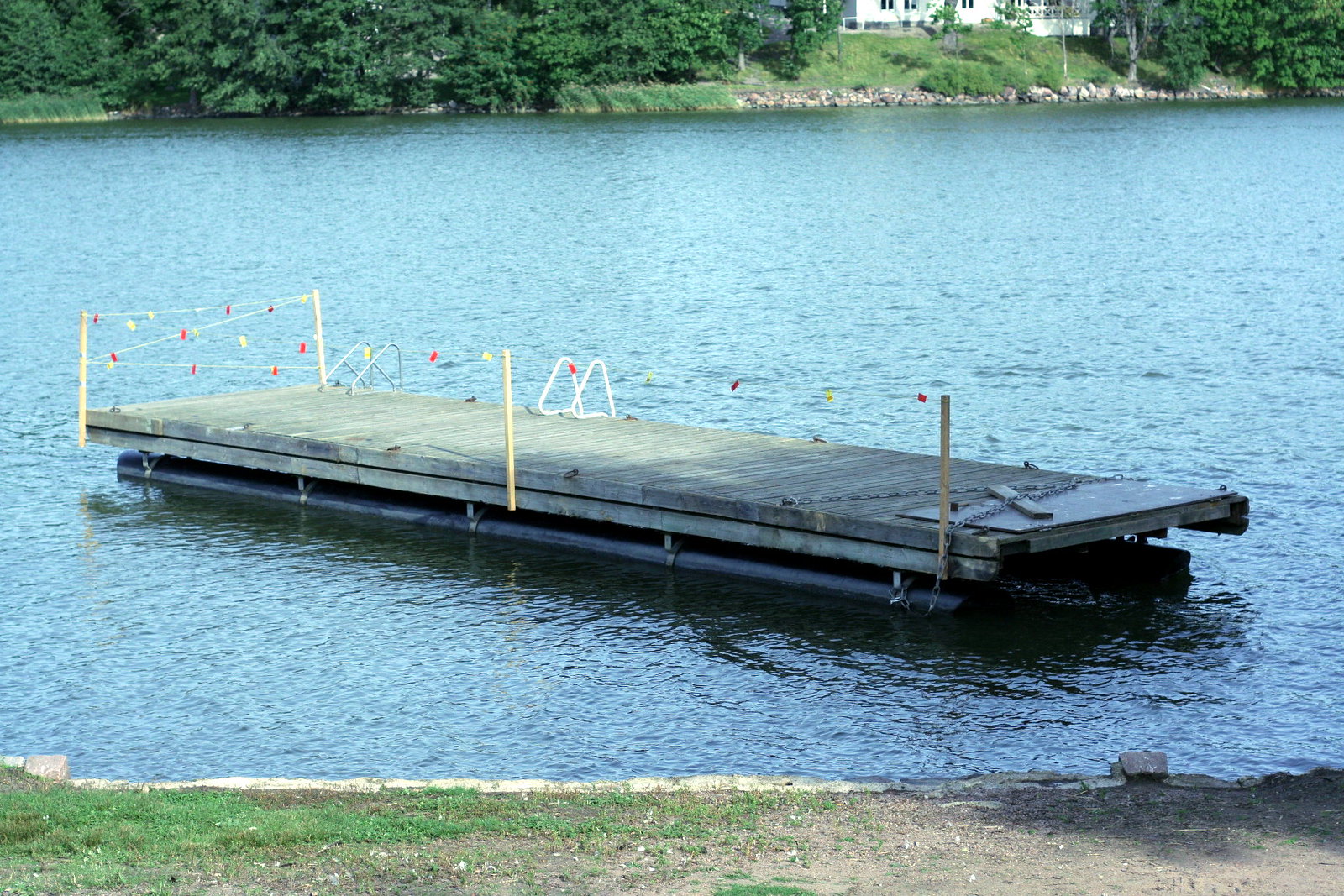The image depicts an outdoor setting by a decently large body of water, likely taken around midday. In the foreground, the ground is patchy with areas of grass and bald spots revealing dirt. Positioned almost directly in the center of the water is a barge or platform, which is angled diagonally to the shore and situated approximately 15 feet from the edge. The platform is equipped with a couple of ladders extending into the water and is decorated with strings of flags.

Across the water, there is a shoreline lined with trees, rocks, and a short hill. Atop the hill, a building or house is visible in the distance. The overall scene features an array of colors including green, brown, gray, white, red, and yellow, accentuating the natural elements and the barge. The tranquility of the setting is heightened by the absence of any textual elements within the image.